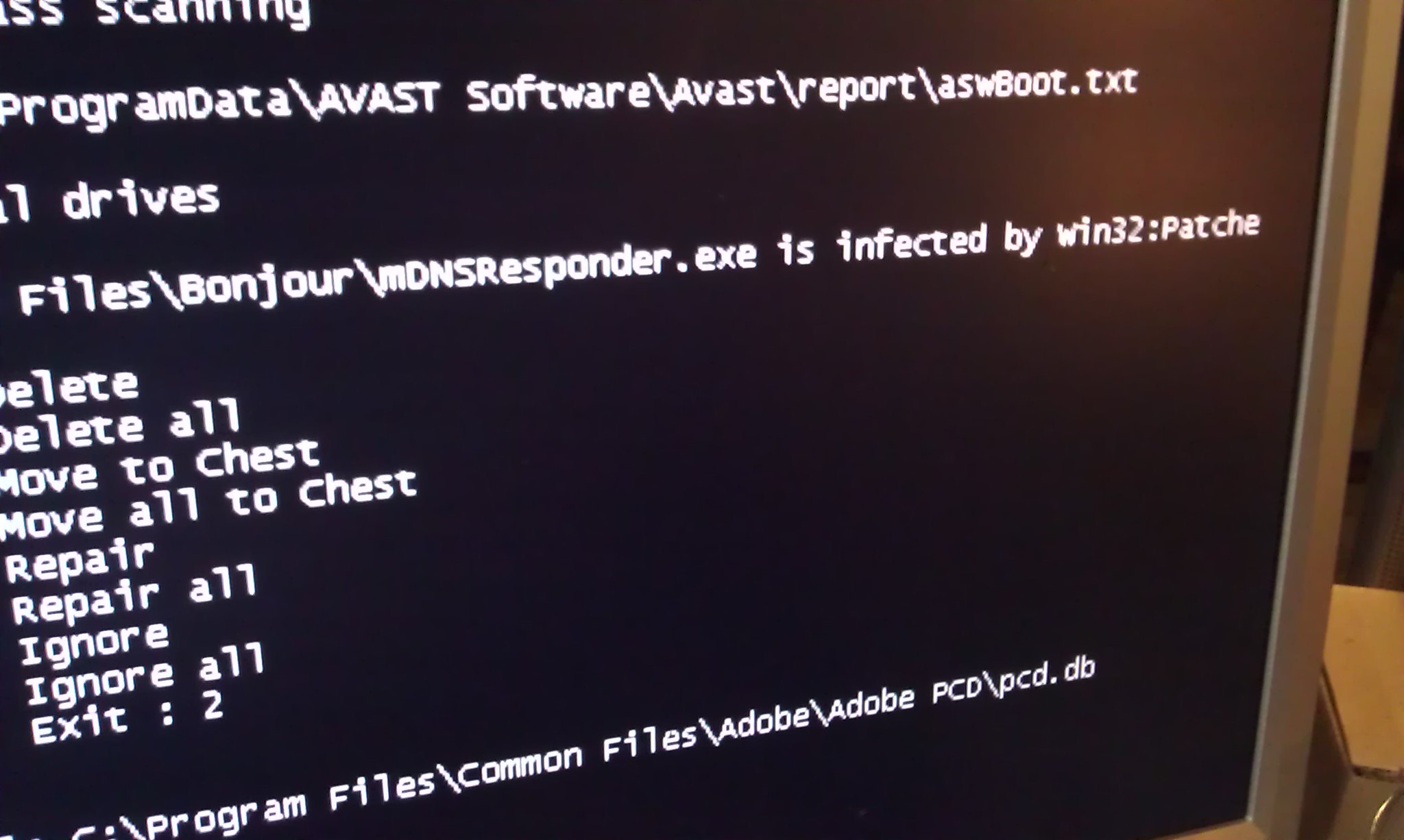The photograph captures a computer screen displaying a diagnostic or antivirus report with a black background and white text. Prominently, it shows a file path detailing various components, including "program data\Avast Software\Avast\report\aswboot.txt drives," indicating it’s possibly related to Avast antivirus software. Below, it reads, "file\bonjour\mdnsresponder.exe is infected by Win32:Patch-e." Further down, there are options listed for handling the infected file: "delete," "delete all," "move to chest," "move all to chest," "repair," "repair all," "ignore," "ignore all," and "exit." At the very bottom, a line partly cut off reads, "C:\program files\common files\Adobe\Adobe PCD\PCD.DB." The edges of the monitor reveal part of a wooden surface on the right and a cardboard box in the bottom corner, confirming this is a photograph of a physical screen rather than a screenshot.